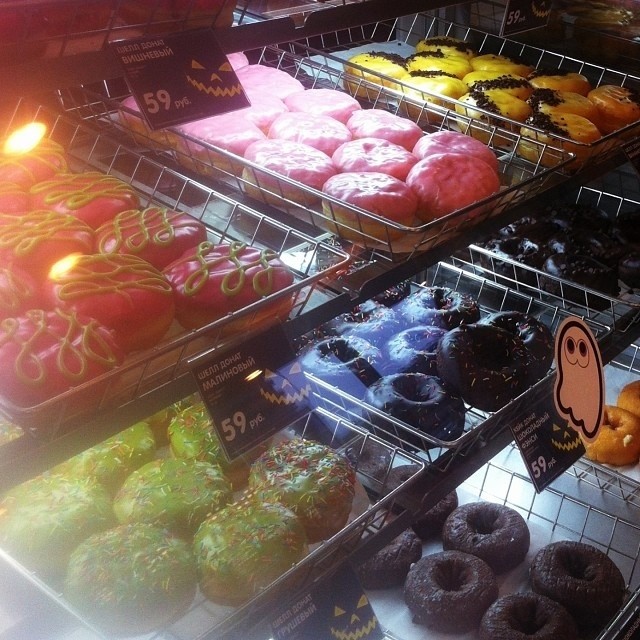This square-shaped, realistic photograph captures the interior of a bakery or grocery store, prominently featuring a glass display case with a reflective surface. Inside the display, there are three rows of metal trays, each filled with an array of donuts, many bearing Halloween-themed decorations. On the top row, we see donuts with vibrant pink frosting, some adorned with yellow or black decorations. These intricate designs include swirling green patterns possibly representing spider webs. The middle row showcases donuts with bright yellow icing speckled with sprinkles, and others with intriguing black frosting which might depict bats. The bottom row is filled with more donuts, coated in rich black chocolate, which add to the spooky theme. Each row has black price cards adorned with a jack-o'-lantern icon, marked with the number 59 in white font, though additional text appears in a different language, rendering it unreadable. The festive decorations, including jack-o'-lanterns and possibly a ghost image, enhance the Halloween ambiance of this well-organized display.